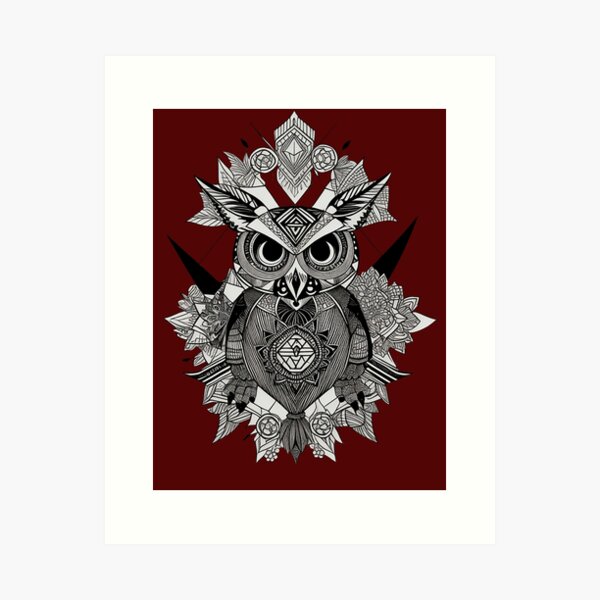The artwork features a striking depiction of a symmetrical, forward-facing owl set against a dark crimson background. The owl itself is rendered in intricate black and white detail, giving it a metallic, almost silver appearance. Its piercing, mean-looking eyes are predominantly black with crescent-shaped white highlights at the bottom. The owl's body is adorned with a variety of ornate patterns, including diamond shapes and floral designs that sprout from its center and extend outward. Additional floral and spiky triangular patterns jut from either side of the owl, contributing to a semi-symmetrical composition. The owl appears to wear a headdress-like structure made of converging half-diamonds and circles at the top. This detailed and psychedelic depiction is framed by a white border on a gray backdrop, enhancing the visual impact of the elaborate design.